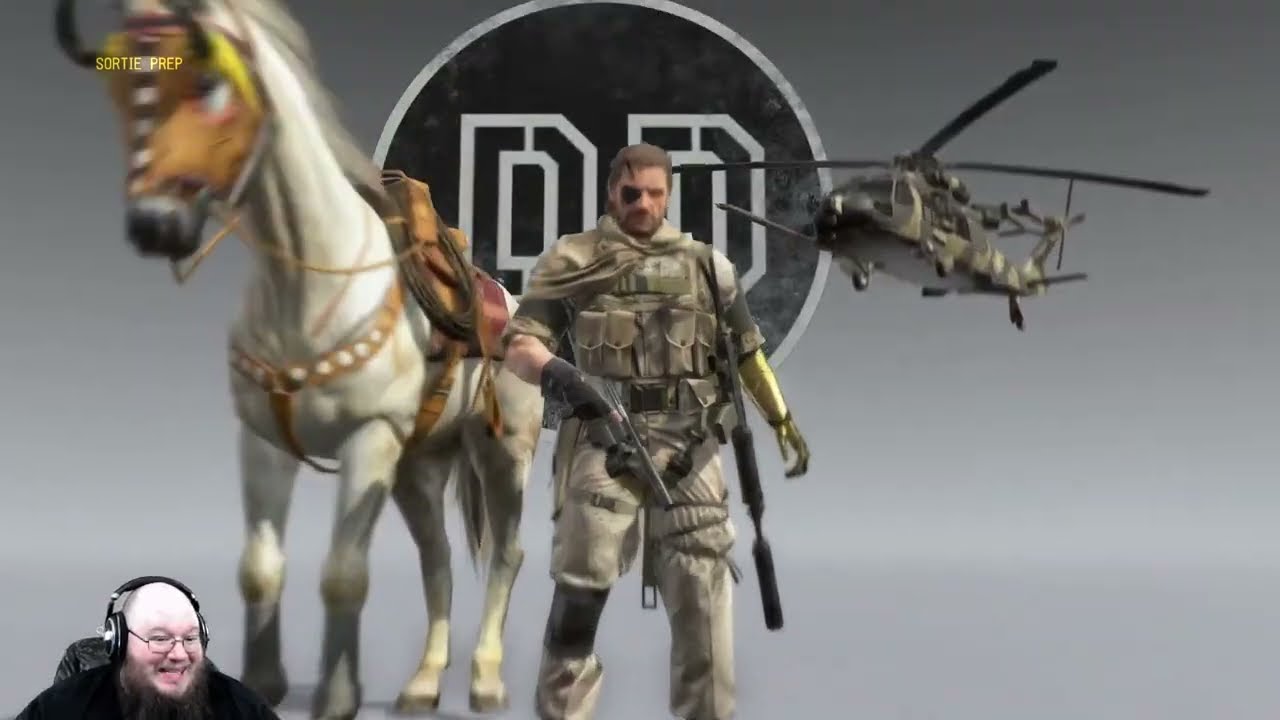The image appears to be a screenshot from a video game interface featuring a heavily armed character and a viewer's live feed in the corner. The background is predominantly grey with a large, somewhat indecipherable oval logo, possibly displaying the letters "DD." At the center, a soldier in tactical gear, including a black eyepatch, a prosthetic arm, and various weapons, stands prominently. He's equipped with a gun in hand and a camo outfit, complemented by gauntlets, a tool belt, and potentially a cape. To the left of the screen, a battle-ready white horse is visible, adorned with a saddle, armor, and a distinctive leather face mask with horns. An army helicopter can be seen in the background. In the bottom left corner, a bald, heavyset Caucasian man wearing glasses, headphones, a dark shirt, and a mustache with a goatee, smiles broadly as he appears to engage with the game, looking either into the camera or at the screen.